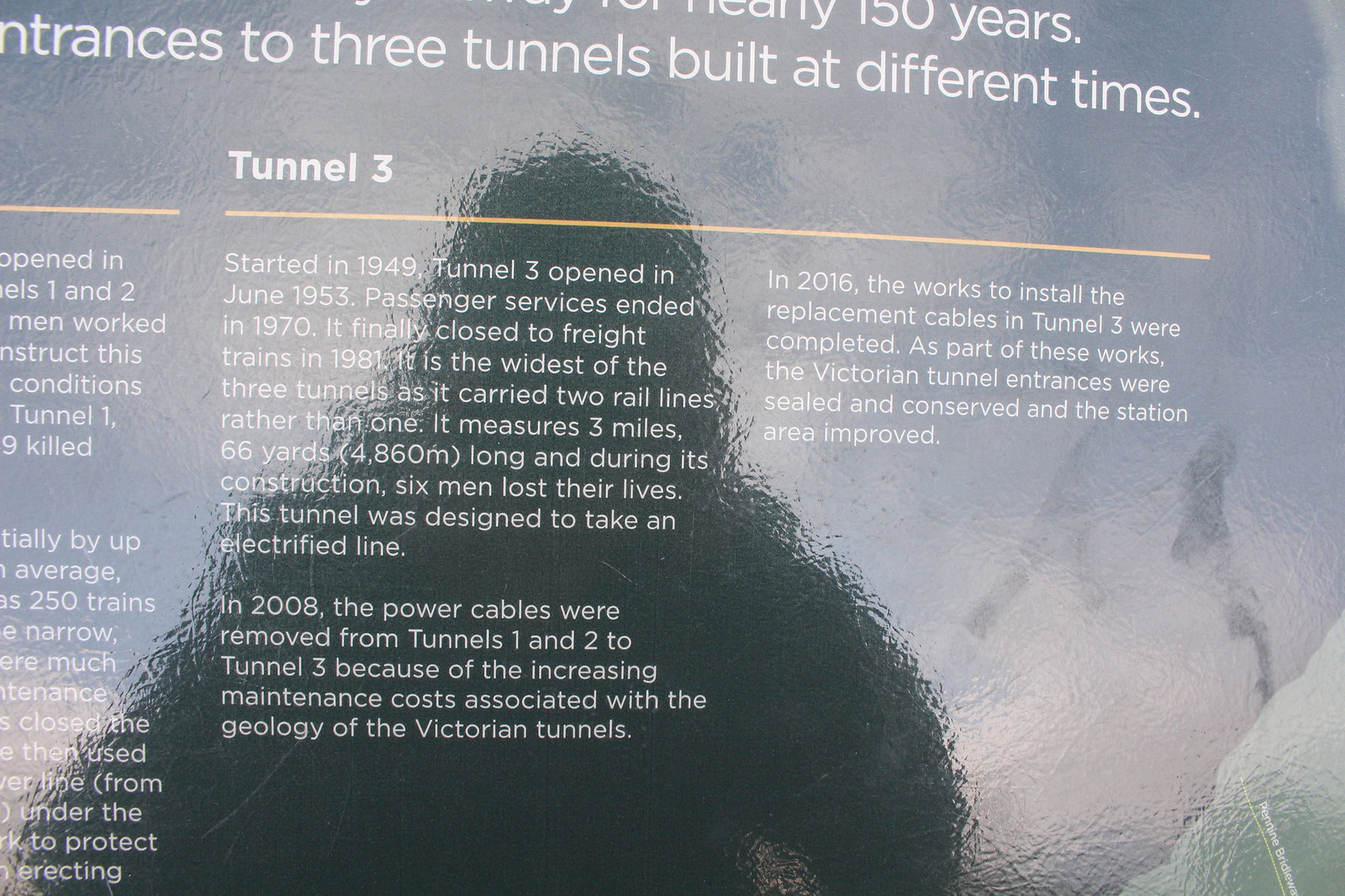The image is a close-up photograph of a dark green sign, part of which is obscured by the reflection of sunlight and the person taking the photograph. The title at the top of the sign is partially cut off. The readable portions indicate the sign is nearly 150 years old and describes the entrances to three tunnels built at different times. Prominently featured in the center of the sign is the title "Tunnel 3" in white, underlined by a yellow horizontal line. The sign details that Tunnel 3 construction began in 1949 and it opened in June 1953. It was the widest of the three tunnels, accommodating two rail lines instead of one, and measured 3.66 miles long. The tunnel ceased passenger services in 1970 and closed to freight trains in 1981. During its construction, six men lost their lives. Additionally, the sign notes that the tunnel was designed to support an electrified rail line. On the right side of the sign, it mentions that in 2016, replacement cable works in Tunnel V were completed. The presence of this sign suggests it might be part of a museum or historical exhibit documenting the history and structural details of these tunnels.